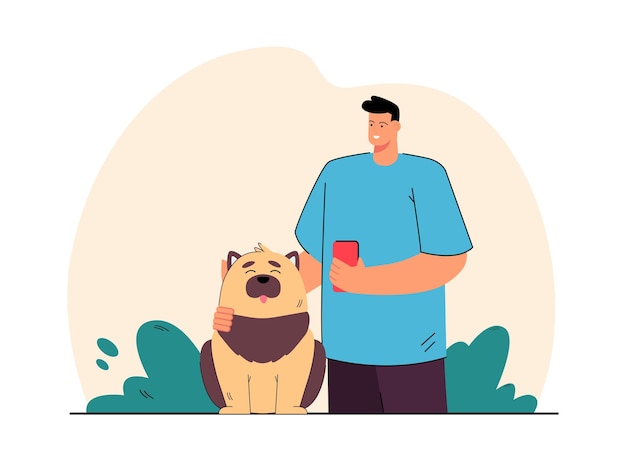This image is an illustration featuring a man and his dog against a light tan background. The man, with a large body and a disproportionately small head, has short black hair, tan skin, and is smiling broadly, revealing his white teeth and black eyebrows. He is dressed in a blue short-sleeved shirt and black shorts and is holding a red cell phone in his left hand. His right arm is affectionately wrapped around his dog. 

The dog, with light tan fur accented by darker brown on its ears, muzzle, chest, haunches, and hind legs, sits contentedly next to the man. Its eyes are closed, its pink tongue hangs out in a happy expression, and it appears to be enjoying the man's company. They are flanked on either side by green bushes, adding a touch of nature to the scene. The overall background has a clean, simple beige tone, emphasizing the duo's joyful interaction in this somewhat whimsical, childlike artwork.